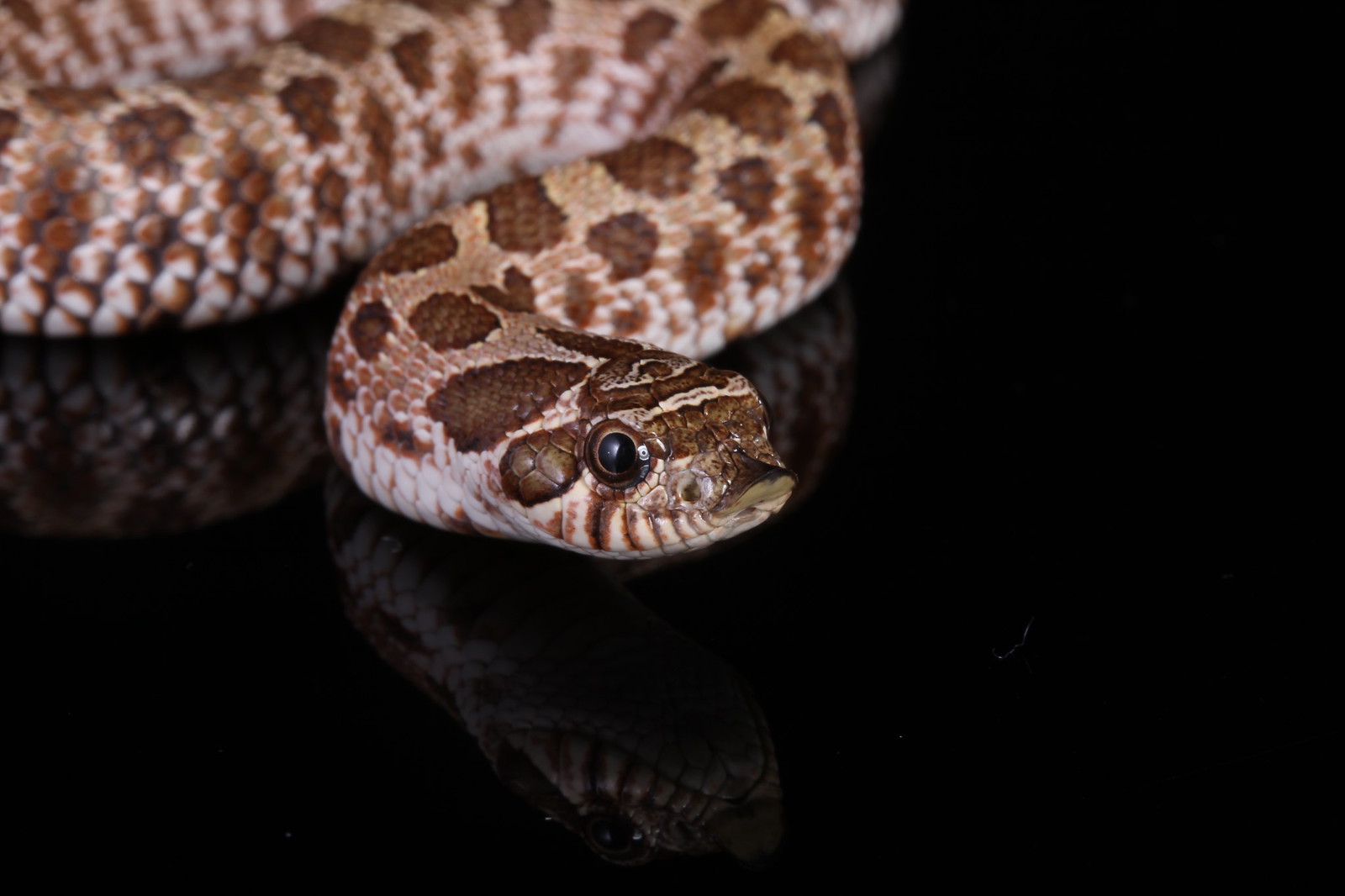The photograph captures a close-up view of a rattlesnake set against a highly reflective, shiny black surface, almost reminiscent of a black mirror. The snake's body, decorated with dark brown patches and a lighter brown hue across the top, is arranged in an undulating pattern, occupying the upper left portion of the image and leading to its head which is meticulously positioned in the center. The head of the snake, with its mouth slightly open, is slightly lifted off the surface, and its front has a distinctive upward slope resembling a short bill. This profile allows for a clear view of one of its very black eyes. The underside scales of the snake appear in a much lighter brown, almost beige color. The surface below is so polished that it casts a striking reflection of the snake, enhancing the visual complexity of the photograph. The background remains entirely black, ensuring that the snake remains the dominant focus of the image.